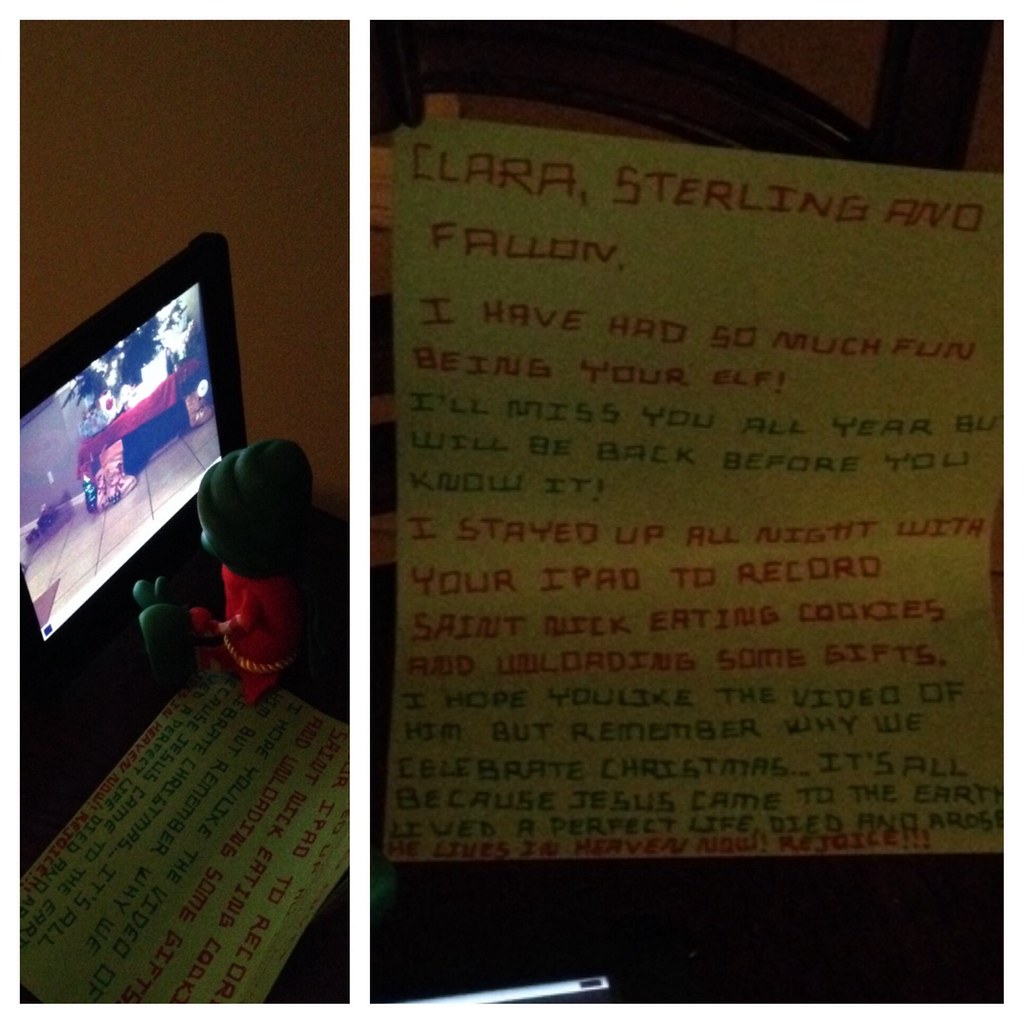The photograph is split into two images. On the left, a small plush toy elf is seated on a yellow piece of paper, intently watching a tablet screen that displays a camera view. On the right, a close-up shot reveals the detailed contents of the note, written in a dark font. The note reads: "Clara Sterling and Fallon, I have had so much fun being your elf. I'll miss you all year, but I'll be back before you know it. I stayed up all night with your iPad to record St. Nick eating cookies and uploading some GIFs. I hope you liked the video of him, but remember why we celebrate Christmas. It's all because Jesus came to the earth, lived a perfect life, died on the cross, and now lives in heaven. Rejoice!" The image features colors such as black, red, white, blue, gray, and green.